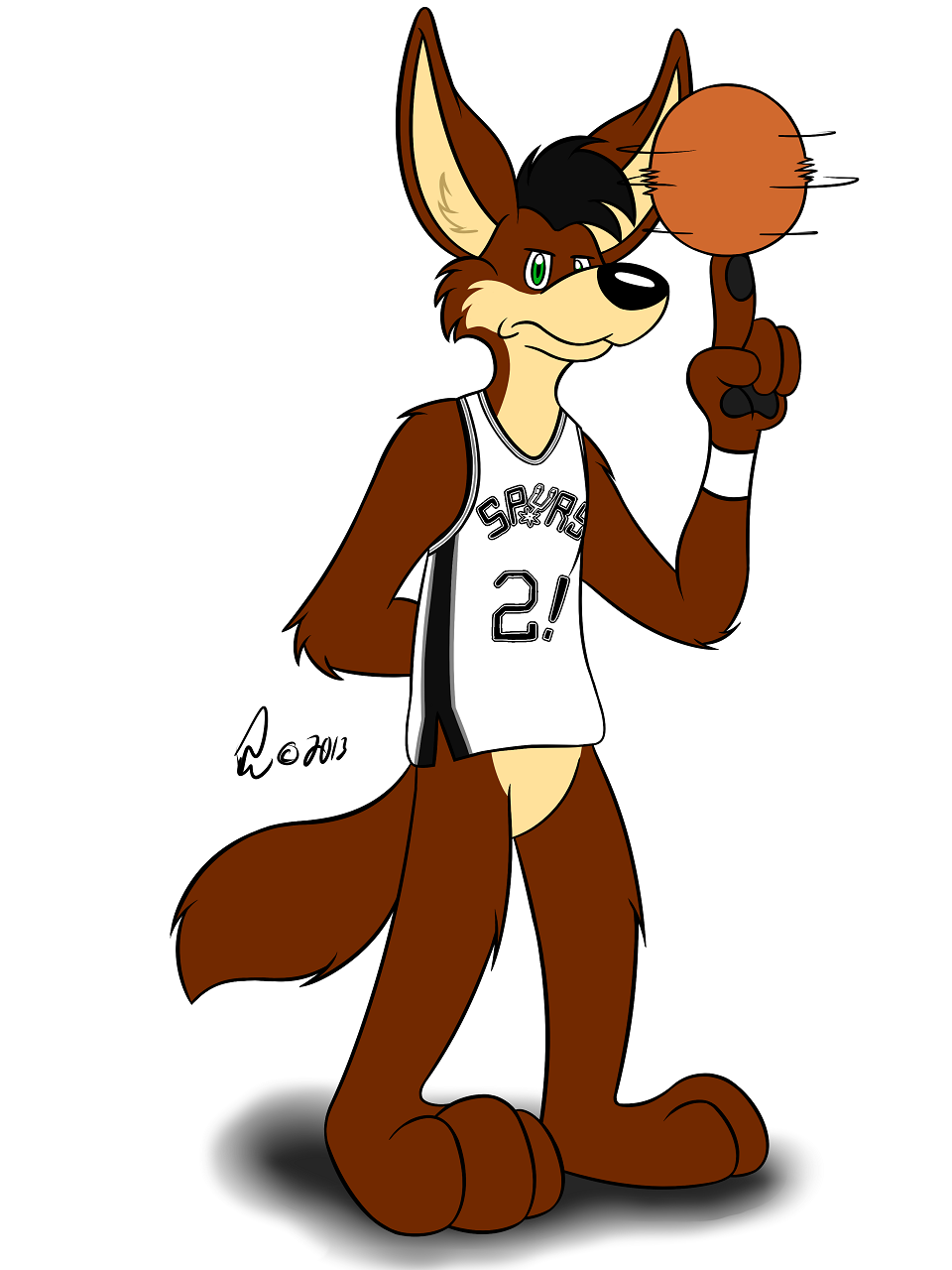The image depicts a cartoon mascot for the NBA team San Antonio Spurs, known as The Coyote. This anthropomorphized coyote is mostly brown with a yellow face and chest, giving the illusion of wearing a yellow outfit. It stands on its hind legs, featuring tall, pointed ears and a tuft of black hair between them. The coyote's left hand is extended, spinning a brown basketball on its index finger, while its right arm is tucked behind its back. Dressed in a black and white basketball jersey with "Spurs" emblazoned on the front and marked with the number "2!" The mascot also has puffy feet and a bushy tail. The drawing includes a partial artist signature, starting with an "R," possibly "Rojo."